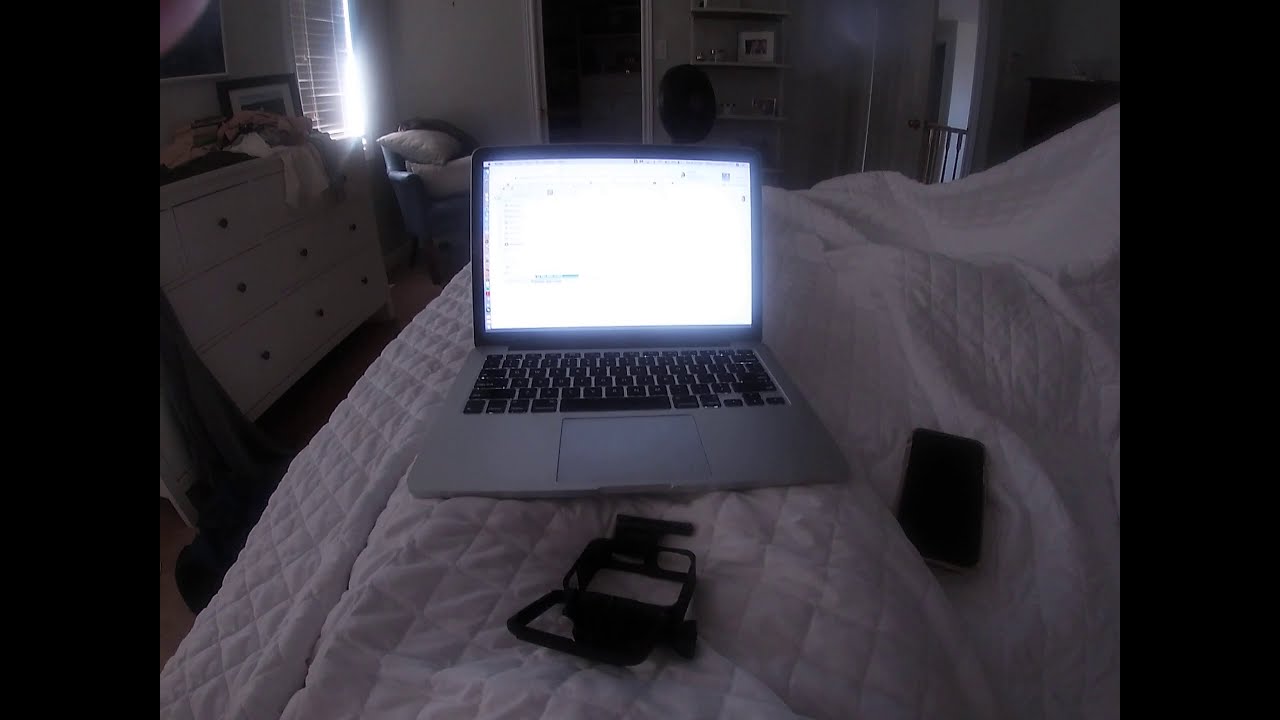In a dimly lit bedroom, a laptop sits on a white, quilted bedspread, its bright screen facing the photographer and casting a glow in the dark room. The bed appears to have a hump, suggesting the presence of someone under the covers, although no person is visible. Scattered around the laptop are a few black objects, possibly a cell phone or similar device. The left side of the room features a dresser cluttered with clothes, and a window with drawn shades, allowing a sliver of sunlight to peek through. Further back, an open doorway reveals a suggestion of stairs or a banister to the right. A chair with pillows is placed in the left corner, next to an open closet door, obscured by darkness. The image is framed with thick black borders on both the left and right sides, adding to the overall shadowy ambiance.